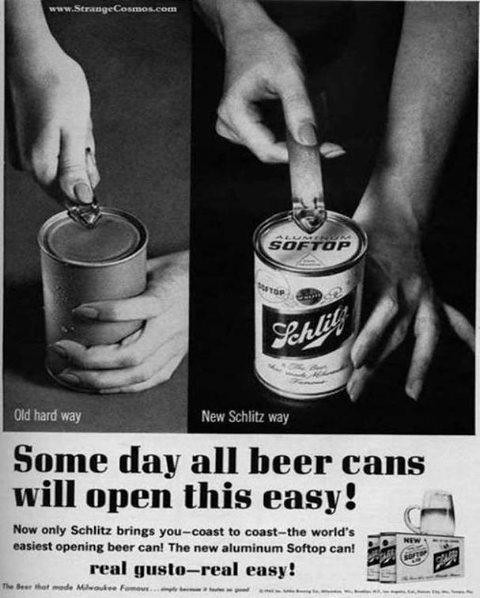This vertical vintage black-and-white advertisement is divided into two main sections. The left side features an old method of opening beer cans, depicted with a photograph of a woman's hand using a manual can opener to open a label-less can against a dark gray background. The label "Old Hardway" is featured at the bottom of this section. The right side showcases the modern Schlitz beer can with an "aluminum soft top," shown in a larger image. This new can is easier to open, as indicated by the "New Schlitz Way" label at the bottom. In the bottom third of the poster, there's a light gray background with bold black text that reads, "Someday all beer cans will open this easy! Now only Schlitz brings you coast to coast the world's easiest opening beer can, the new aluminum soft top can. Real gusto, real easy." Additionally, an image in the lower right corner displays a box of Schlitz beer with a half-filled mug on top. The top of the ad features the website www.strangecosmos.com.